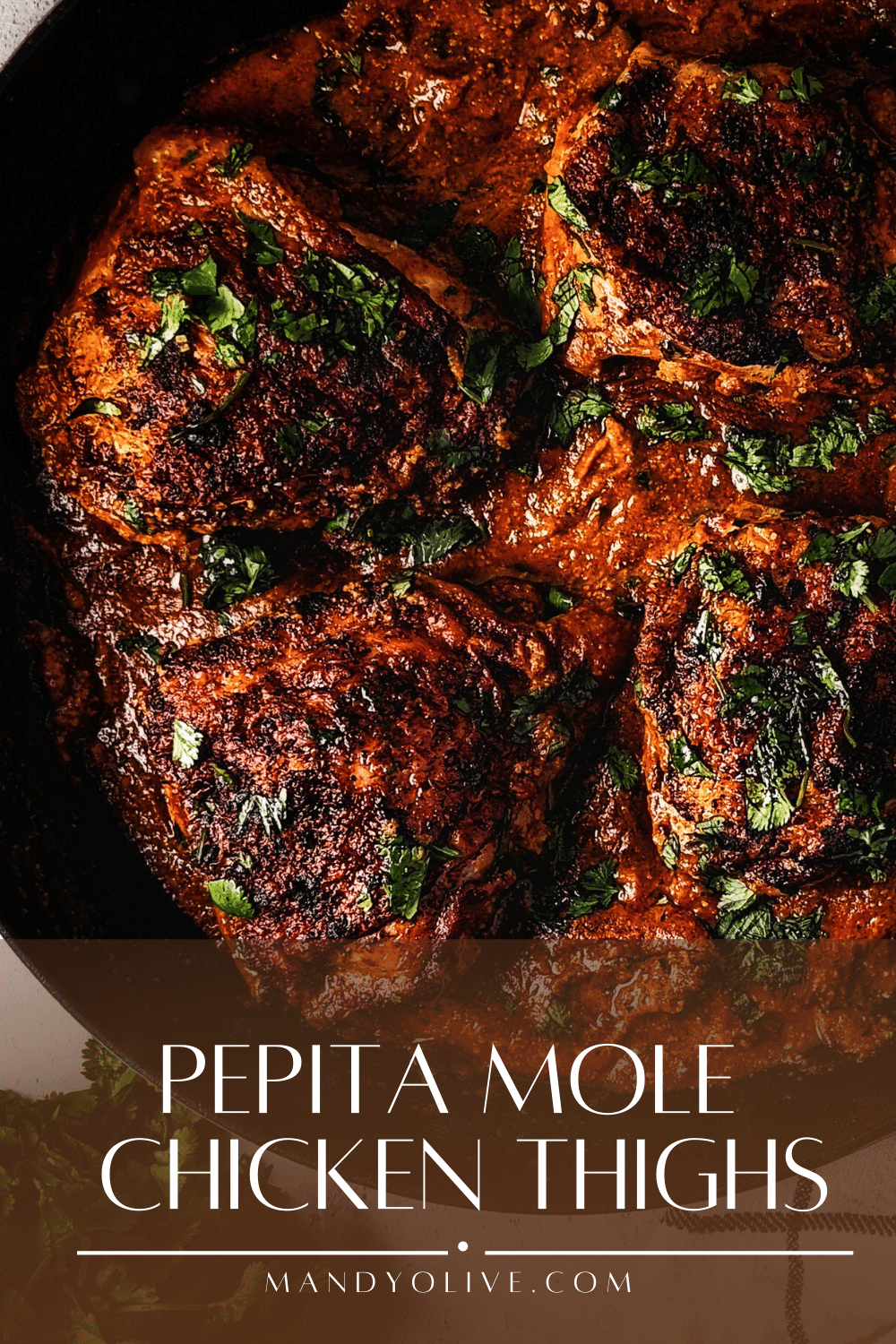This vertically-oriented image showcases a close-up of perfectly cooked chicken thighs, arranged side-by-side. The chicken thighs are adorned with a dark, reddish-brown, caramelized coating, possibly indicating a rich and savory mole sauce. Small green leafy herbs are embedded into the coating, adding a touch of freshness and color contrast. At the bottom of the image, bold white text, in all capital letters, reads “PEPITA MOLE CHICKEN THIGHS.” Directly below this, a small white circle is depicted with two horizontal white lines beneath it, indicating the brand or website. Beneath this icon, the text "mandyolive.com" is displayed, suggesting that this image serves as an enticing advertisement for this particular recipe, driving viewers to visit Mandy Olive’s culinary website for more details.